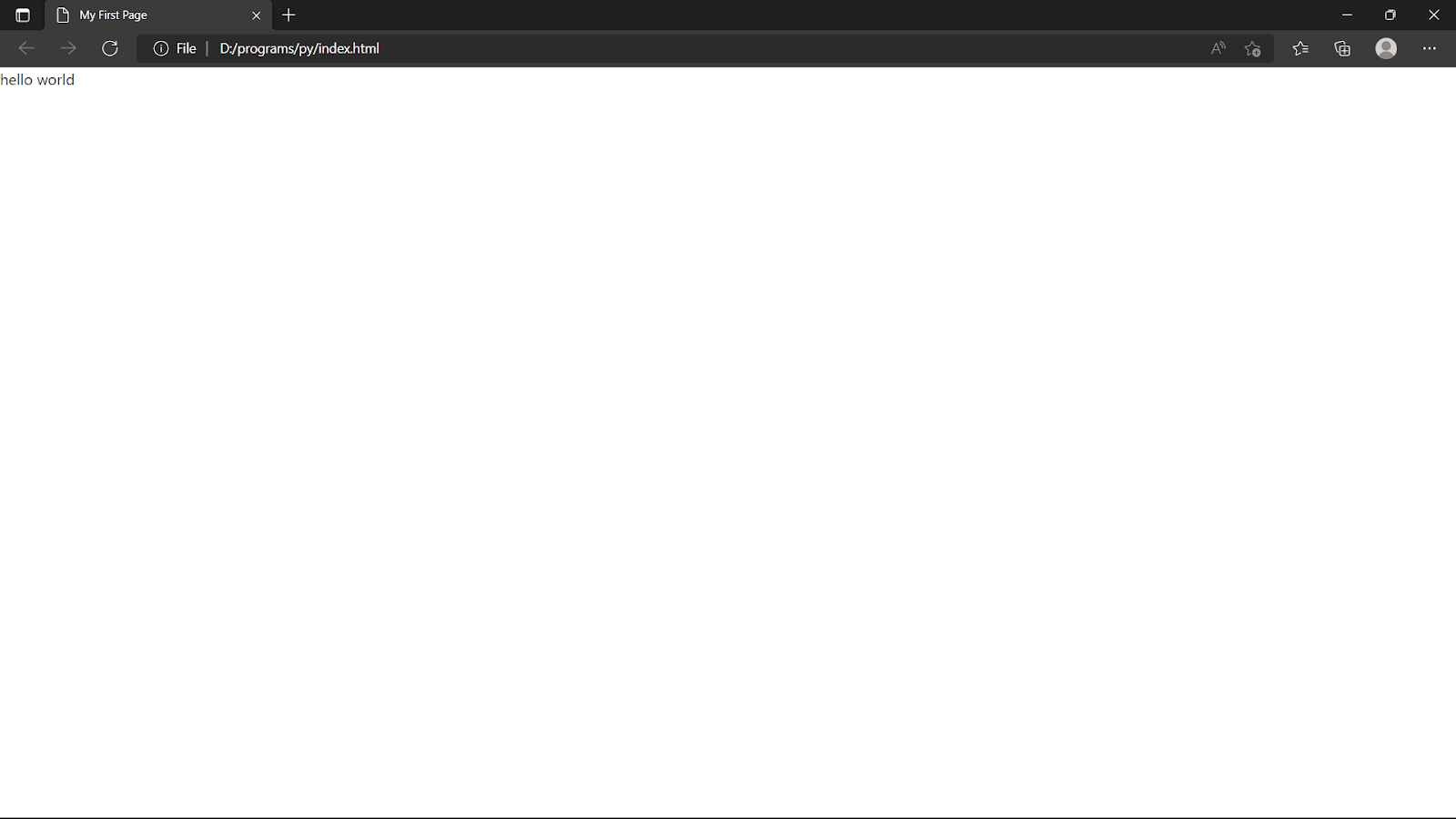The image captures a rectangular, blank white page displayed on a computer monitor, possibly from a PC or laptop. At the top of the screen is a charcoal gray navigation bar. In the upper left corner, there's a square white icon resembling a grid, which opens a menu. To the right of this icon is a tab labeled "My First Page," accompanied by a paper icon on its left. Adjacent to the tab on its far right is a white 'X' symbol for closing the tab, while to the right of this tab on the gray bar is a plus sign for opening new tabs.

Below the navigation bar is a slightly lighter gray toolbar, featuring a back arrow, a forward arrow, and a white circle for reloading the page. To the right of these icons is the text "File." The URL bar displays "D:/programs/py/index.html."

At the very top of the white section, the text "hello world" is written in lowercase black lettering. On the far right of the screen, several additional icons are visible: an 'X' to close the window, a profile icon, a tabs icon, a star indicating the number of bookmarks, and a font size adjustment icon.